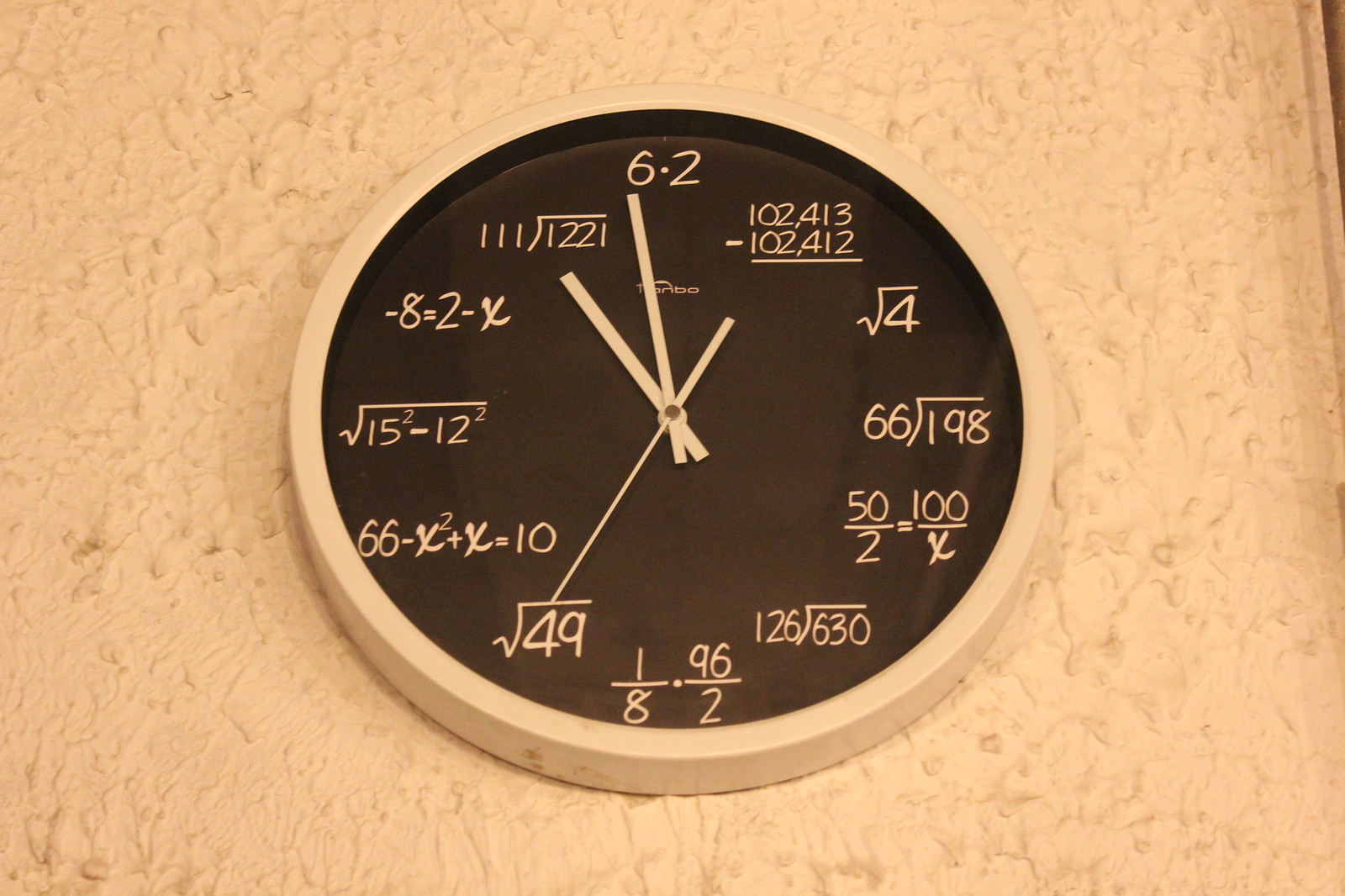This image features a highly unique and intellectually stimulating clock, where every hour is represented not by ordinary numerals, but by intricate mathematical equations. For instance, the number 12 is denoted by the simple multiplication equation 6 * 2. The number 1 is expressed as the result of 102,413 minus 102,412. The number 2 is represented by the square root of 4. These equations span a fascinating range of mathematical concepts, including division problems, fractions, algebraic equations involving solving for x, and numerous square roots and powers. Each equation is meticulously crafted to yield the hour it symbolizes, creating an engaging and educational experience for anyone who reads the clock.